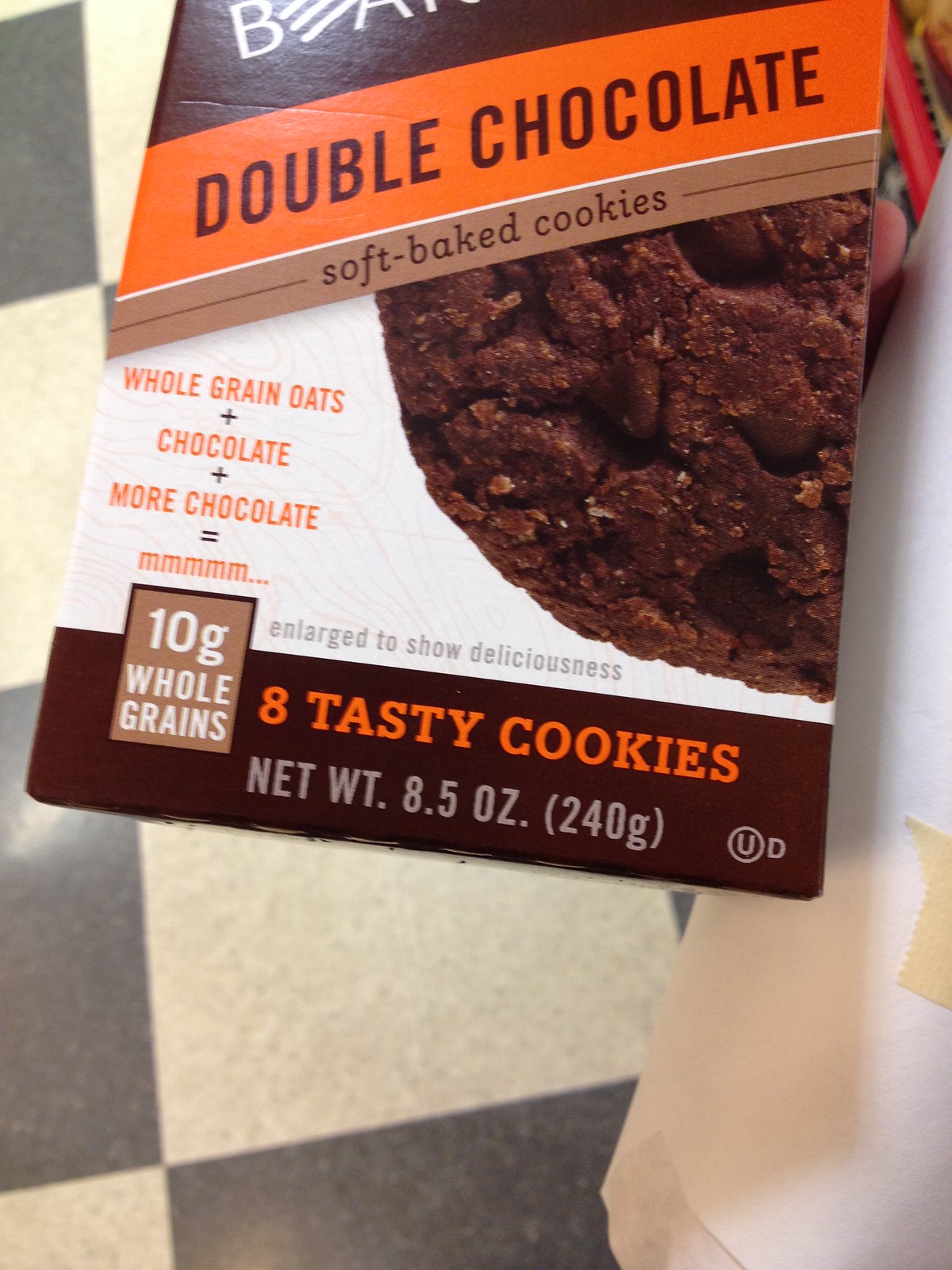The photograph features a package of food against a checkerboard-style floor composed of black and white speckled tiles. The white tiles exhibit a gray speckled pattern, while the black tiles feature lighter speckles. The packaging itself is primarily brown, featuring an orange stripe with the text "Double Chocolate" in brown. Another brown stripe below reads "Soft Bake Cookies." The package also contains a white section with a subtle wood grain and orange background, displaying the text "Whole Grain Oats + Chocolate + More Chocolate = M-m-m-m-m..." On the right side of the package, there's an image of a dark chocolate cookie. Additional text states "10 Whole Grains Enlarged to Show Deliciousness," alongside a brown strip with orange lettering indicating, "8 Tasty Cookies" and "Net Weight 8.5 oz (240g)."